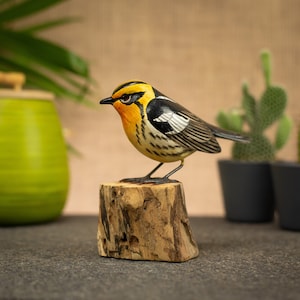The image features a small, intricately detailed bird figurine perched atop a mini tree stump. This figurine is smaller than a four-inch plant pot and stands on a black felted surface. The bird’s head is a golden yellow with a small black beak and a distinctive black stripe running across it. Its back and wings are black with white vertical stripes, while its underbody is white. The bird’s lifelike design and vibrant colors make it the central focus of the image. In the softly lit background, against a beige cream-colored wall, there are a couple of small potted plants—one positioned in the top left corner and another on the right side of the image. The overall image is bright and clear, emphasizing the natural light that enhances the details of the figurine and surrounding elements. However, the slightly grainy texture suggests it might not be a real bird but rather a meticulously crafted statue.